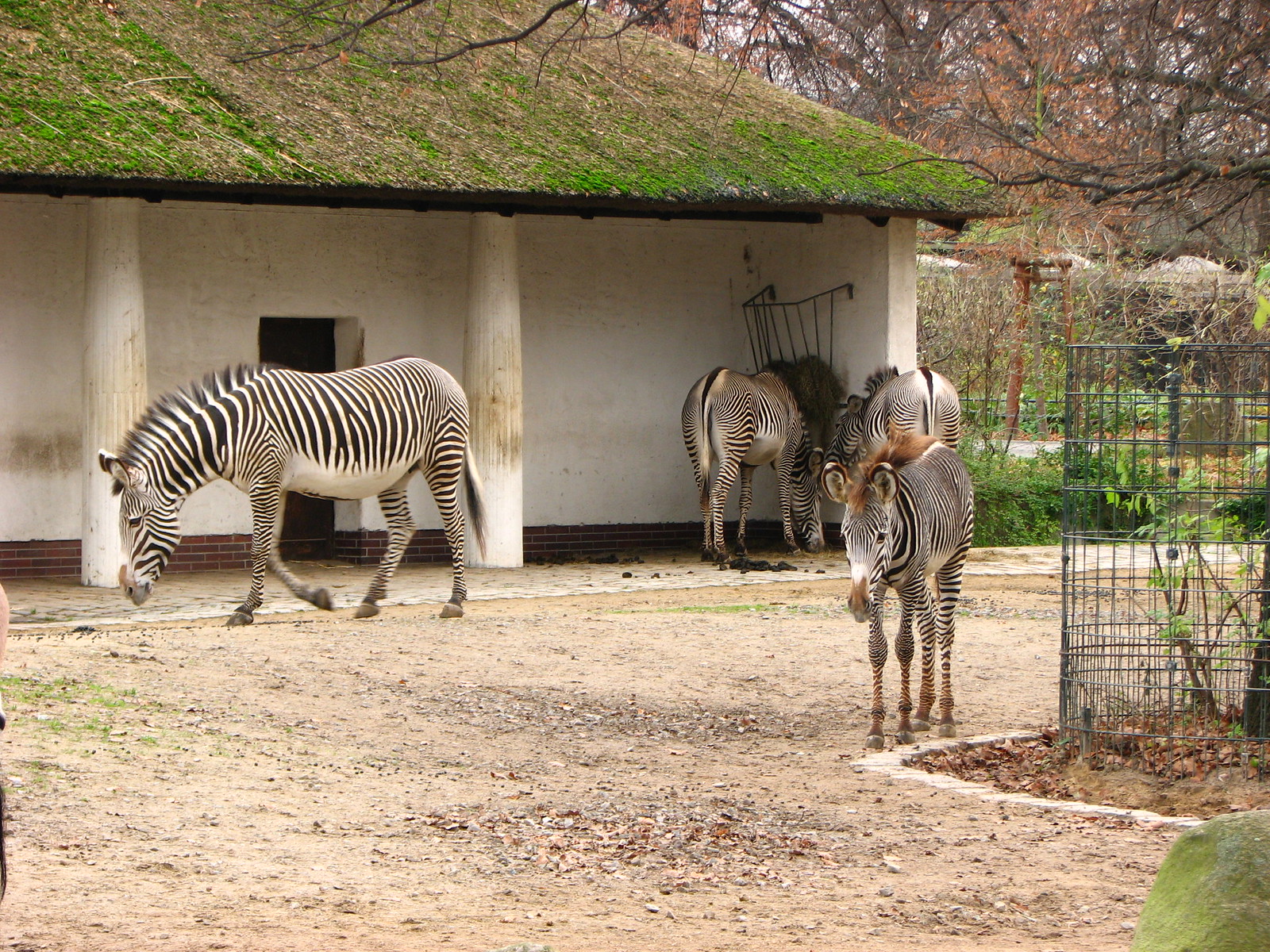In this image, captured likely at a zoo, there are four zebras in a courtyard setting. The scene features an adult zebra on the left, with its head down, facing left and appearing to be in motion. This zebra is distinguished by its size and posture. To the right of this zebra and towards the center, you find another two adult zebras in the background, both with their heads down, seemingly feeding from a hay rack attached to the wall of a white barn with brick layers and dark spots where zebras have rubbed against it. The hay rack is filled with hay. 

The focal point of the image is a smaller, baby zebra positioned on the right side, near a metal cage surrounding a bush. This young zebra stands out due to its reddish-brown hair flowing through the middle of its ears and similarly colored, slender legs. It faces almost directly towards the camera, drawing attention with its unique coloring. 

The background features a partially open white barn with a moss and dry leaf-covered roof and a reinforced open doorway. The courtyard floor consists of brown dirt and sand, with patches of grass and shrubbery, including a tree with red leaves and bushes. There is a black fence along the right side, and a small, rock-strewn garden area protected by a wire cage adds to the scenery. This detailed setting suggests a well-thought environment aimed at mimicking a natural savannah habitat, complete with greenery and various architectural elements.